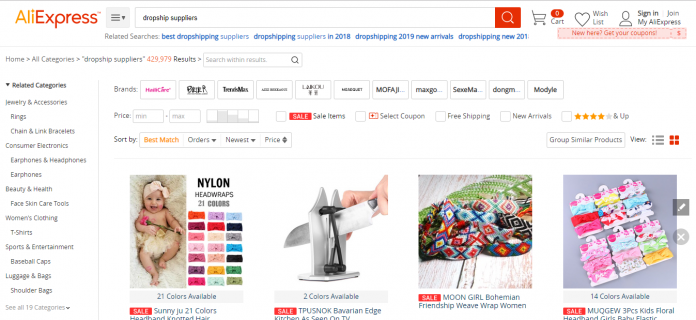This webpage screenshot from AliExpress features a comprehensive layout geared towards drop shipping suppliers. The top-left corner prominently displays the AliExpress logo in bold red. Centralized at the top, the text "Drop Ship Suppliers" is featured. On the top-right corner, there are icons and links for the shopping cart, wish list, sign-in, and a join area.

Beneath the main title, on the left-hand side, there are navigation columns with links labeled Home, All Categories, Drop Ship Suppliers, and Results. Situated further down on the left side are vertical columns under "Related Categories," listing sectors such as Jewelry and Accessories, Rings, Chain and Link Bracelets, Consumer Electronics, Earphones and Headphones, Earphones, Beauty and Health, Face Skin Care Tools, Women's Clothing, T-Shirts, Sports and Entertainment, Baseball Caps, Luggage and Bags, Shoulder Bags, and a link to see all 19 categories.

The center section features filtering options, allowing users to input minimum and maximum price ranges, check items on sale, select coupons, choose Free Shipping, New Arrivals, and rate products by star ratings. Below these filters, sorting options are available for Best Match, Orders, Newest, Price, and Grouping Similar Products.

A gallery of product images is displayed underneath. Featured items include a baby modeling nylon head wraps in various colors, a knife sharpener honing a large knife, Bohemian Friendship Weave Wraps for Women, and Kids Floral Headbands for Girls in numerous colors.